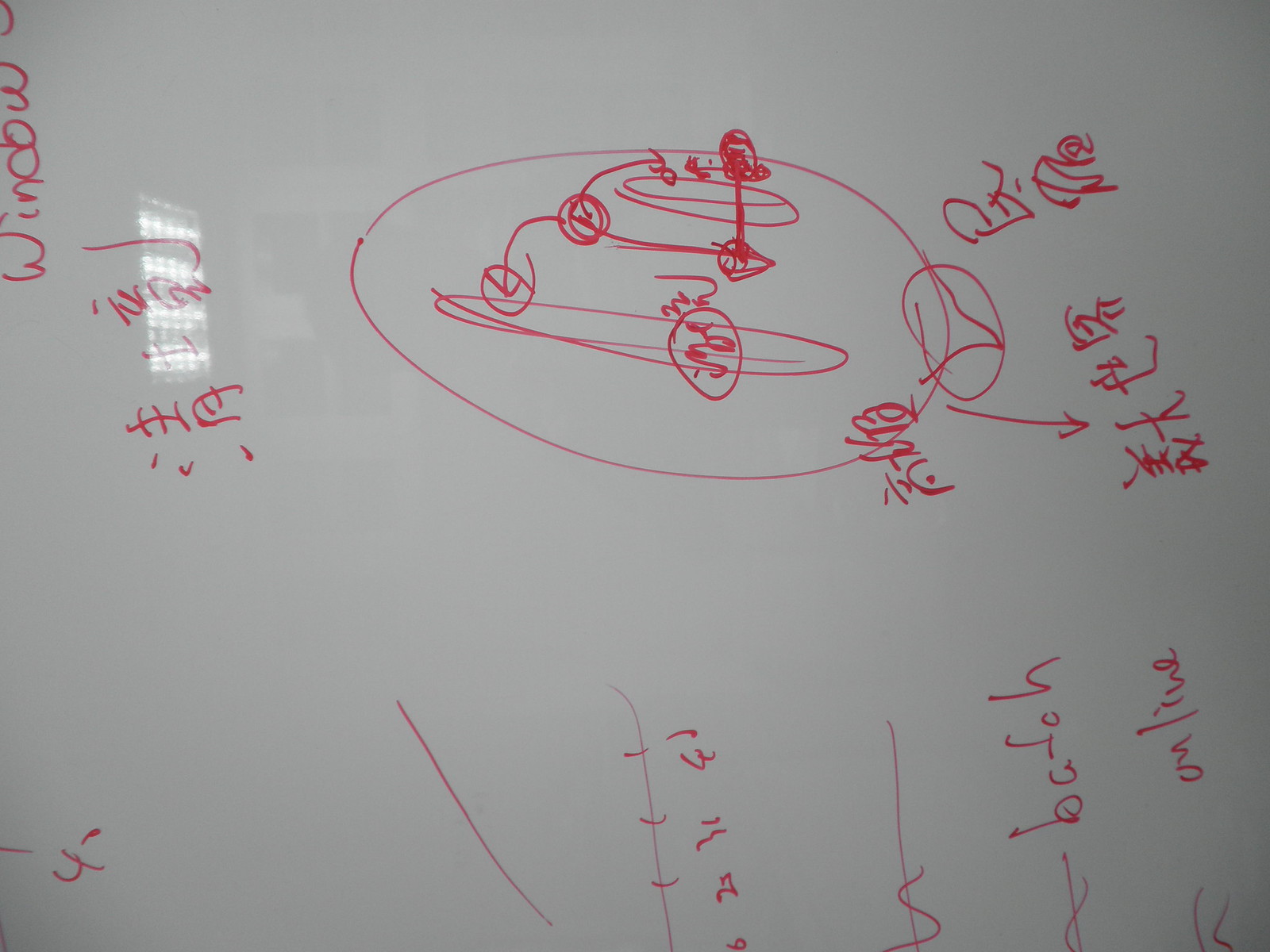This image captures a whiteboard with a reflective glare, likely from a window seen in the top left corner. The board is filled with various inscriptions and is positioned sideways. Turning the image to the right reveals a mix of Asian characters and English text. Prominently, there is a large circle with numerous scribblings at the top of the photo, reminiscent of something being crossed out or a dense cluster of notes. To the left, a bar graph is visible with numerical values including 20, 30, and a mysteriously incongruent 61. In addition to the visuals, an English word "batch" is noted at the bottom, and the word "window" along with the digit "4" can be discerned at the top right when the image is properly oriented.